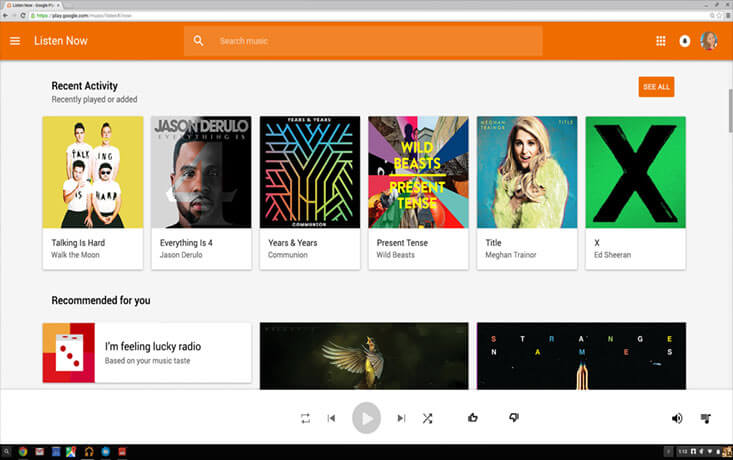Here is a detailed, cleaned-up caption for the described image:

"The image showcases a digital interface with a clean white background and an orange header labeled 'Listen Now' accompanied by a ember icon. Below, a search bar is prominently displayed. The interface is divided into six squares arranged in two rows of three, likely representing different content sections. On the upper right corner, there's a profile icon featuring a picture of a lady and a section titled 'Recent Activity' that highlights 'Recently Played or Added' items. 

One of the highlighted entries is titled 'Talking is Hard' by a group of four members. Each member's shirt displays a part of the phrase: 'Talk,' 'ing,' 'is,' and 'hard.' Another entry features Jason Derulo with the notable number '4,' and a song titled 'Everything is 4.' Additionally, a colorful, maze-like design in rainbow hues is linked with the artist 'Years and Years,' depicting various images of people and buildings.

Another recommended piece is 'Wild Beasts - Present Tense,' showing a lady in a green jacket. There's also a green square with a black 'X' titled 'Title.' At the bottom of the interface, there is a section labeled 'Recommended for You,' with 'I'm Feeling Lucky Radio based on your music taste.'"